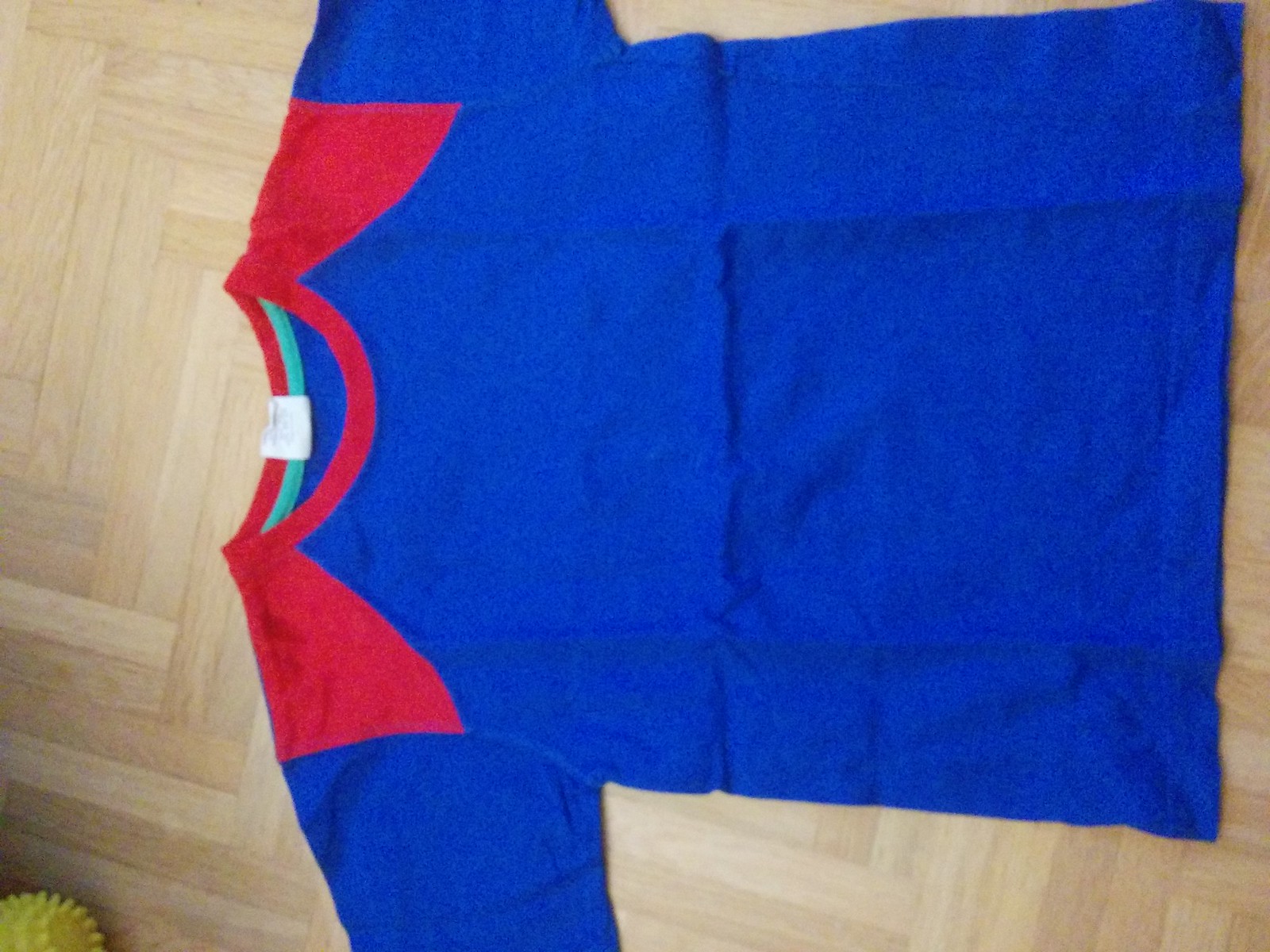The image features a color photograph taken indoors of a shirt laid flat on a light wood inlaid floor. The shirt, which appears to have just been unfolded given the visible crease marks, is a bright navy blue with a red crew neck collar and matching red patches extending onto the shoulders. Inside the neckline, a light blue or aqua stripe is visible beneath the red trim, accompanied by a white tag that likely contains standard garment information. In the bottom left-hand corner of the image, there is a yellow spiky ball, possibly a pet toy, adding an additional element of interest to the composition.